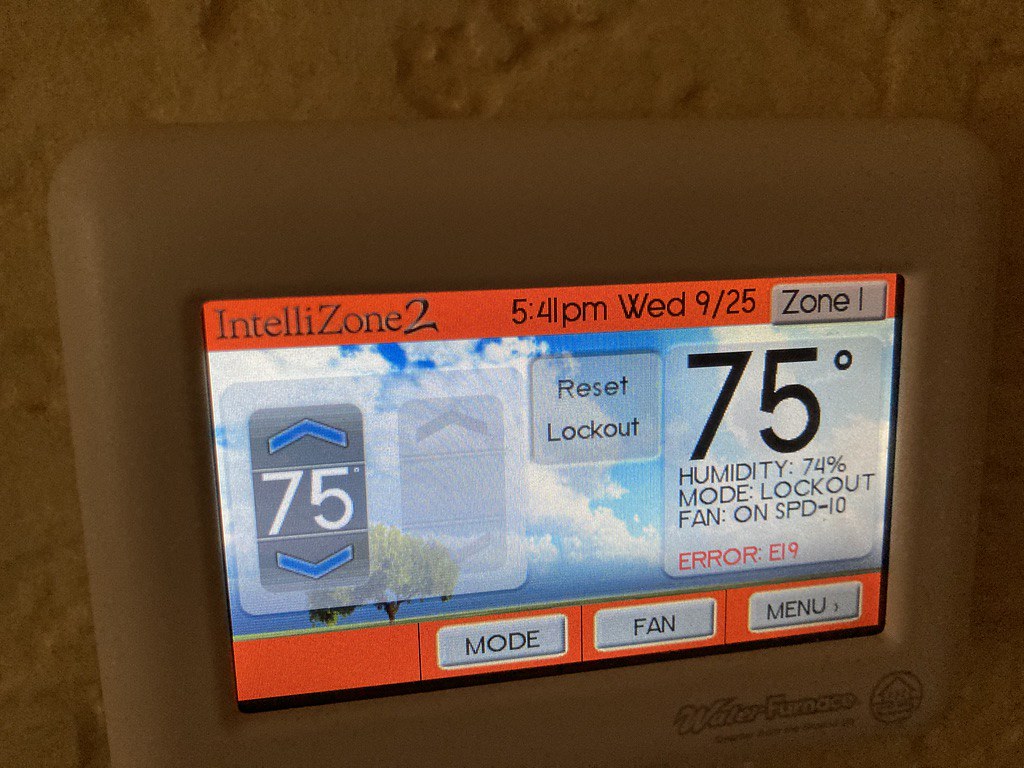This photograph captures a detailed view of a control panel display, affixed to a stone-effect beige wall. The image appears to be taken indoors under low-light conditions, without the use of flash, and relies on a light source emanating from the left side. The control panel itself is framed by an outer plastic border in a cream or beige hue.

At the bottom right of the unit's border, the text "WaterFurnace" is visible alongside a circle logo featuring a house, followed by company details. The digital display is full-color, brightly illuminated, and detailed.

At the top of the screen, there is a red horizontal stripe with the text "IntelliZone 2" in black, along with the current time "5:41 p.m.," the day "Wednesday," and the date "9.25." Adjacent to this information is "Zone 1" displayed in gray.

The main area of the display features a serene image of a blue sky with white fluffy clouds and a green tree. An opaque square overlay shows the temperature "75" with up and down arrow options for adjustment. Below this, a darker gray-transparent block reads "reset or lockout."

On the right side of the display screen, large opaque blocks contain further information: the temperature "75 degrees," humidity at "74%," "mode: lockout," "fan: on," and "speed: 10." Notably, in red text, an "error E19" message is displayed.

At the bottom of the display is an orange line, beneath which are three gray rectangular buttons labeled "mode," "fan," and "menu." 

This intricate setup suggests a sophisticated and user-friendly control panel interface designed for precise environmental regulation within a residential or commercial setting.